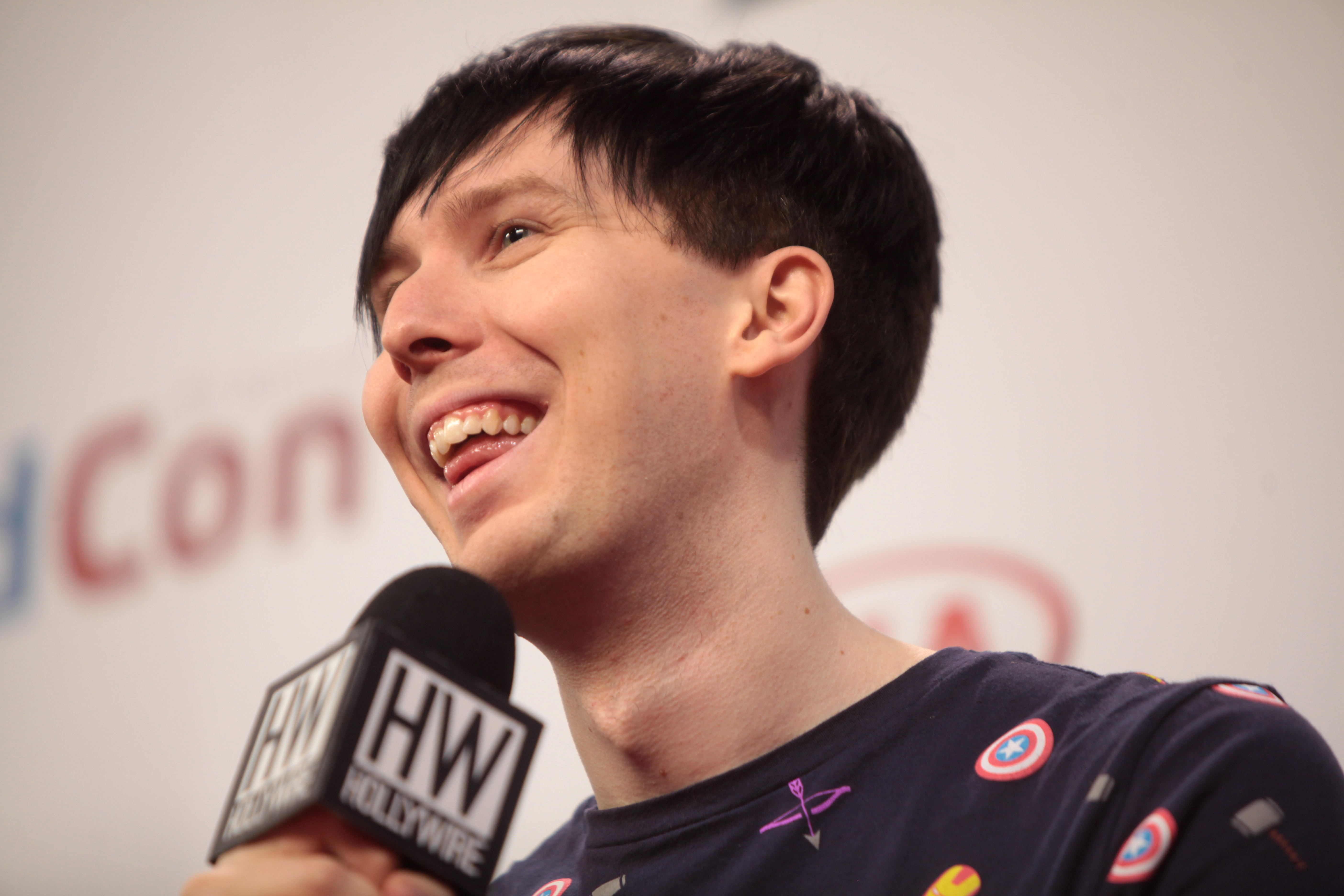This horizontally aligned rectangular close-up photograph captures Phil Lester at a comic convention, noticeable by the blurred white wall in the background with the partially visible letters "CON" in red. Phil is facing to the left and slightly forward, sporting a silly smile with his mouth open, showing his top teeth and tongue. His medium-length dark hair includes bangs that fall slightly forward. Phil is holding a black microphone with a white square section beneath the tip, which is labeled with "HW" and "Hollywire" underneath. He is wearing a dark-colored T-shirt, either black or dark blue, adorned with various small symbols including elements related to Captain America. The image reflects a lively moment, possibly during an interview or a panel discussion at the event.